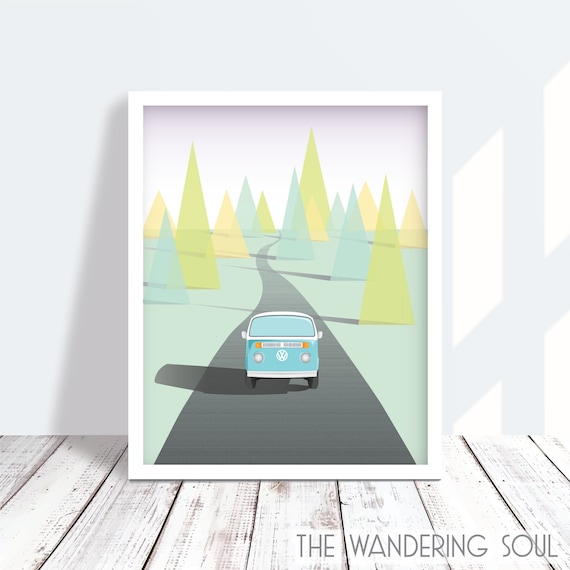The image features a highly stylized and artificial-looking painting, leaning against a white wall on a wooden plank floor. The painting, appearing almost computer-generated, depicts a light blue Volkswagen bus driving towards the viewer on a long, slightly curved road. The scene presents a forest area with trees represented by geometrical triangular shapes in various colors, including blue and orange. The background of the painting merges into the context of a larger artwork, making the frame's boundaries ambiguous. The shadow on the right side of the frame appears unnatural and may symbolize a window or other elements in a stylized manner similar to the trees. The entire composition includes soft hues of light yellow, green, blue-teal, black, off-white, gray, and a subtle light pink in the sky. At the bottom of the painting, the text reads "The Wandering Soul."